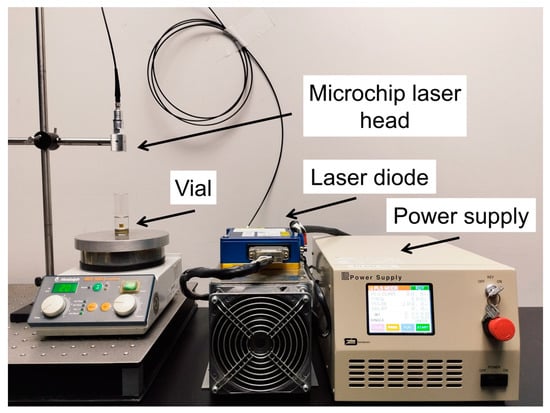This is a detailed color photograph taken indoors, likely in a science classroom or work center, showcasing a labeled diagram of various electronic components involved in a scientific process, possibly related to a microchip laser system. The equipment is neatly arranged on a black table against a beige wall. Each primary component in the image is clearly labeled with text and arrows indicating specific items. On the left, a label points to a "vial" placed on top of what resembles a measuring scale, featuring several buttons and a display. Adjacent to the vial is the "microchip laser head," identified as part of a thin, pole-like structure likely integral to the laser assembly. Central to the photograph is a blue box labeled "laser diode," characterized by a fan-like structure with circular imprints, indicative of cooling components. To the right side of the image sits a substantial tan-colored, rectangular box labeled "power supply." This box has a screen with colored indicators at the top and bottom, a key switch, a red button, and additional vented fan areas. The overall image is softly hued with pastel tones, giving it an older, slightly retro appearance. This detailed equipment diagram provides insight into the sophisticated arrangement and labeling necessary for scientific experimentation with microchip laser systems.